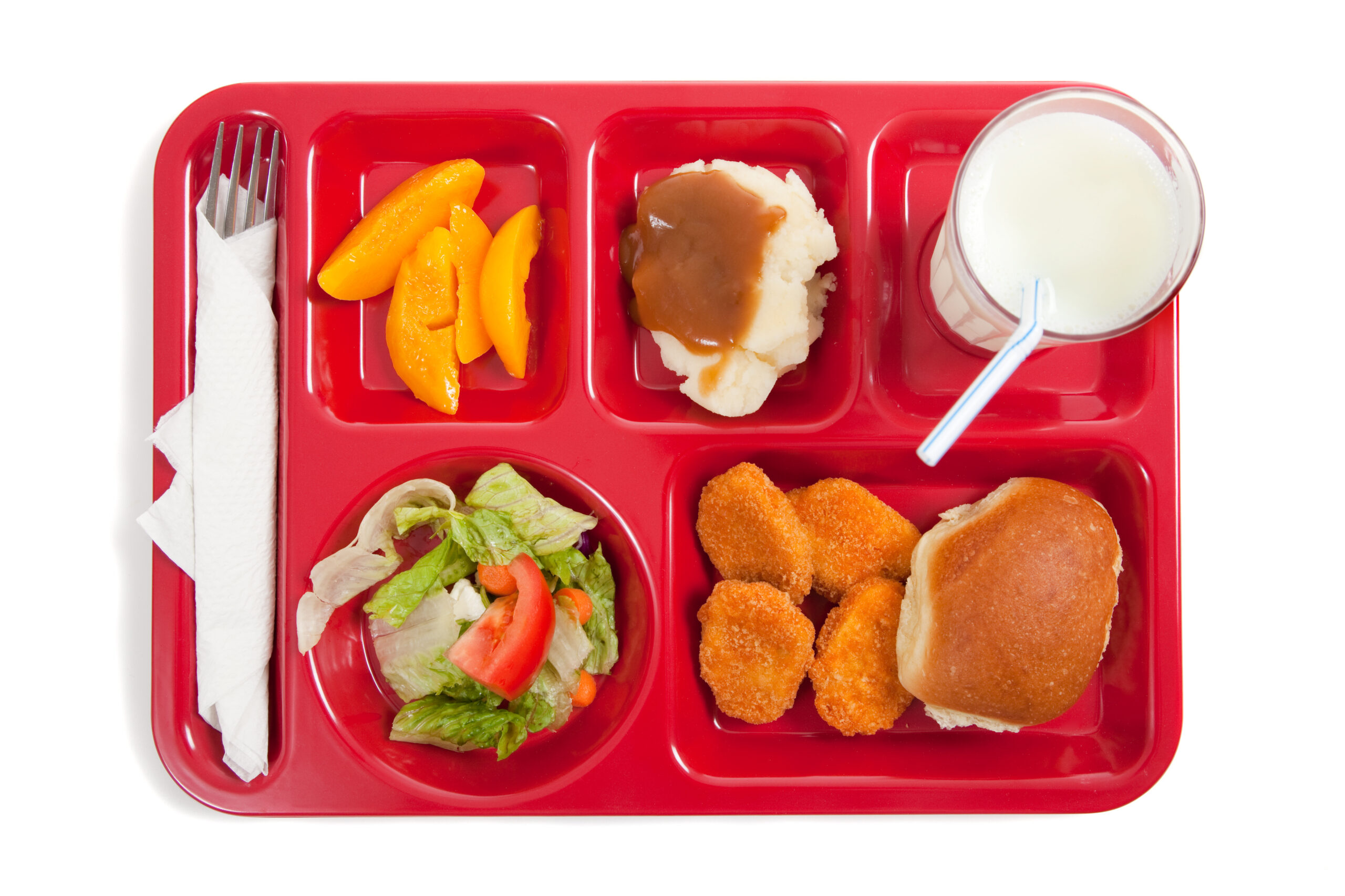This overhead close-up photo features a bright, shiny red school cafeteria tray with a total of six compartments. On the left side of the tray, there is a white napkin-wrapped fork. The upper-left compartment contains several slices of yellow peach. The middle top compartment is filled with creamy white mashed potatoes covered in brown gravy. The upper-right compartment holds a cup of white milk with a blue-striped straw emerging from it. The bottom-left, round compartment showcases a fresh green salad, which includes pieces of lettuce, red tomato, and bits of carrot. The largest, rectangular compartment on the bottom right houses four golden-brown chicken nuggets and a small round bun. The overall layout and variety of foods contribute to a typical school lunch setting.